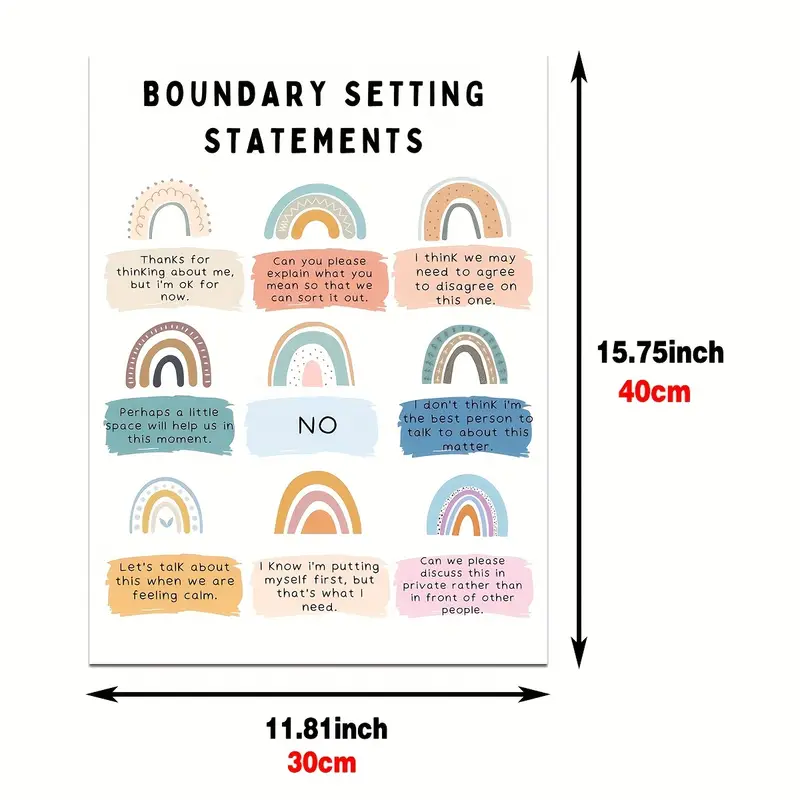The image is a detailed safety flyer meant for children, possibly from a teacher, focused on setting boundaries. It features a vertical rectangular white sheet measuring 15.75 inches (40 centimeters) tall, as indicated by a black double-headed arrow on the right side, and 11.81 inches (30 centimeters) wide, as shown by a black double-headed arrow at the bottom. The title "Boundary Setting Statements" is centered at the top in black text. Below the title, there are three rows of three pastel-colored rainbows in various shades of oranges, purples, browns, and blacks, each occupying a square segment. Underneath each rainbow, there is a rectangular paint streak in a matching pastel color and a corresponding statement in black text, aimed at teaching respectful communication and personal boundaries. The statements include:

1. "Thanks for thinking about me, but I'm okay for now."
2. "Can you please explain what you mean so that we can sort it out?"
3. "I think we may need to agree to disagree on this one."
4. "Perhaps a little space would help us at this moment."
5. "No."
6. "I don't think I'm the best person to talk to about this matter."
7. "Let's talk about this when we are feeling calm."
8. "I know I'm putting myself first, but that's what I need."
9. "Can we please discuss this in private rather than in front of other people?"

Each row of rainbows and statements adds up to a 3x3 grid, providing a visually appealing and organized layout for the flyer.